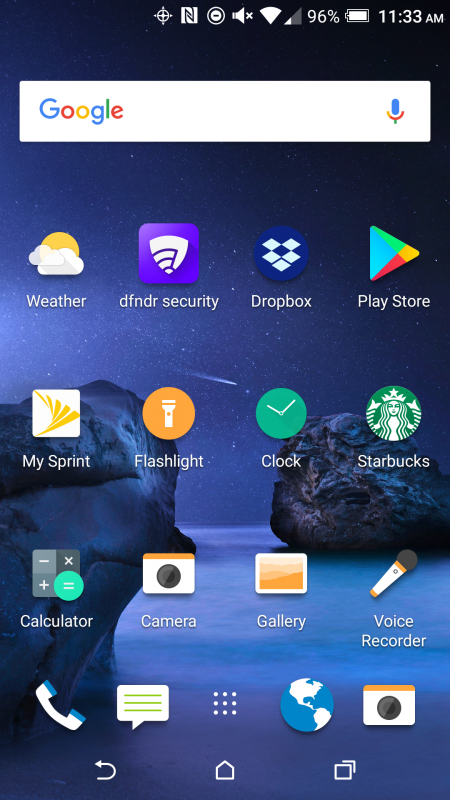The image depicts an Android phone's home screen at night. In the top right corner, several icons are visible, including indicators for wireless signal, cellular connection, and battery life. Below these, there's a search bar with "Google" entered in it, accompanied by a microphone icon on the right.

The background, or screensaver, showcases a serene night scene featuring water and two rocks, one on either side of the image. The home screen is populated with various app icons, each labeled for easy identification.

In the first row of icons, there's:
1. A sun with clouds representing the weather app
2. DFNDR security app
3. Dropbox
4. Play Store

The second row includes:
1. My Sprint
2. Flashlight
3. Clock
4. Starbucks

The third row features:
1. Calculator
2. Camera
3. Gallery
4. Voice Recorder

The fourth row contains additional icons without explanatory text:
1. A white phone icon
2. A speech bubble with lines across it
3. Nine dots arranged in a 3x3 grid
4. An image of a globe
5. A picture of a camera

At the bottom of the screen, there are three navigation icons:
1. An arrow forming a nearly complete circle (typically the refresh or recent apps button)
2. A house icon (home button)
3. Two overlapping squares (task manager or recent apps).